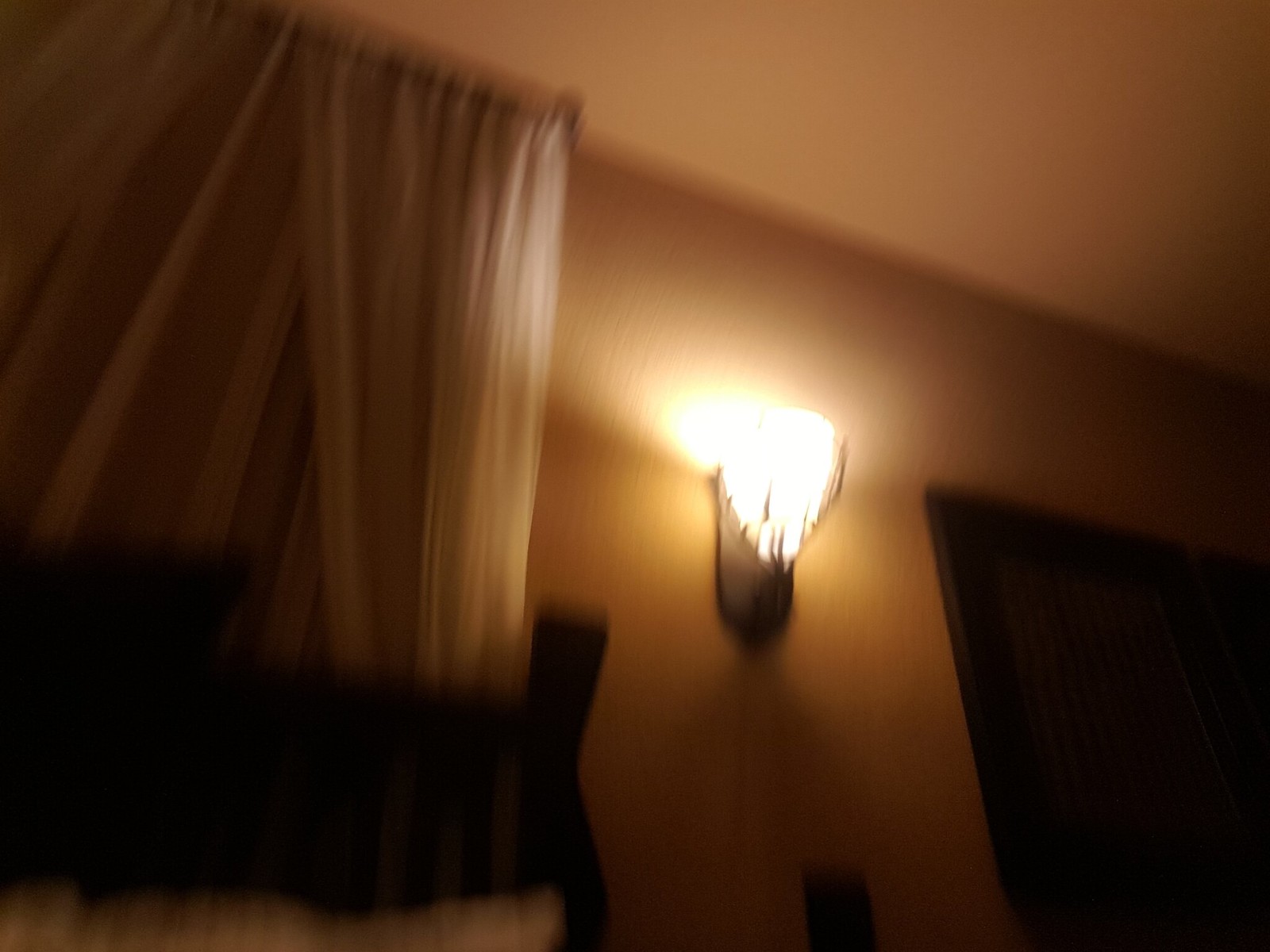The photograph depicts a blurry scene of a bedroom, focused on a portion of the wall. Central to the image is an upward-pointing, Art Deco-style wall sconce, glowing brightly but casting minimal light beyond its immediate vicinity. The sconce features a black, oval-shaped backing and a tiered design reminiscent of an inverted ziggurat. The room's walls appear to be white or beige, though the image's blurriness makes it hard to discern exact colors and details.

To the left of the sconce, sheer white curtains are visible, possibly layered over solid drapes that are pulled to the side. Below the curtains, a partially visible black object, likely the headboard of a bed, is barely detectable. There are some white, soft shapes beneath it that resemble pillows, though they are partially cropped out of the photo.

On the right side of the image, two square brown frames are mounted horizontally on the wall. Below the sconce and towards the bottom right corner, there's a dark square shape, possibly a door, a mirror, or the top of a dresser, though its exact nature remains unclear due to the blurry quality of the photograph.